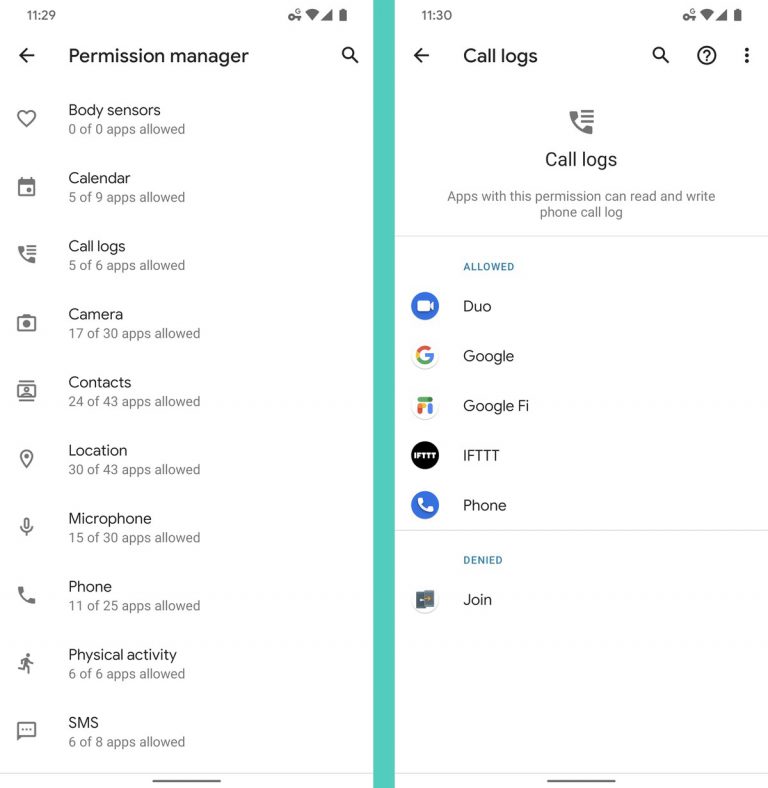This image showcases detailed screenshots of a phone's Permission Manager and Call Logs pages. The phone in question, with screen captures taken on October 29 and 30, shows the device is fully charged, connected to Wi-Fi with full bars.

### Permission Manager
- The background is white, with black text and a search bar positioned on the right side. 
- A back button is located on the left side of the screen.
- **Permissions Breakdown:**
  - **Body Sensors**: 0 of 2 apps allowed (icon: heart)
  - **Calendar**: 5 of 9 apps allowed
  - **Call Logs**: 5 of 6 apps allowed
  - **Camera**: 17 of 30 apps allowed
  - **Contacts**: 24 of 43 apps allowed
  - **Location**: 30 of 43 apps allowed
  - **Microphone**: 15 of 30 apps allowed
  - **Phone**: 11 of 25 apps allowed
  - **Physical Activity**: 6 of 6 apps allowed
  - **SMS**: 6 of 8 apps allowed

### Call Logs Permissions
- This page also includes a back button, search bar, question mark icon, and context menu (three vertical dots) on the far right.
- It indicates that apps with this permission can read and write the phone call logs.
- **Apps with Call Log Permissions:**
  - **Allowed**: Duo, Google, Google Fi, IFTTT, Phone.
  - **Denied**: One unidentified app.

These screenshots reveal extensive apps permissions, particularly those accessing contacts and locations, highlighting the user's openness to granting various apps significant data access.